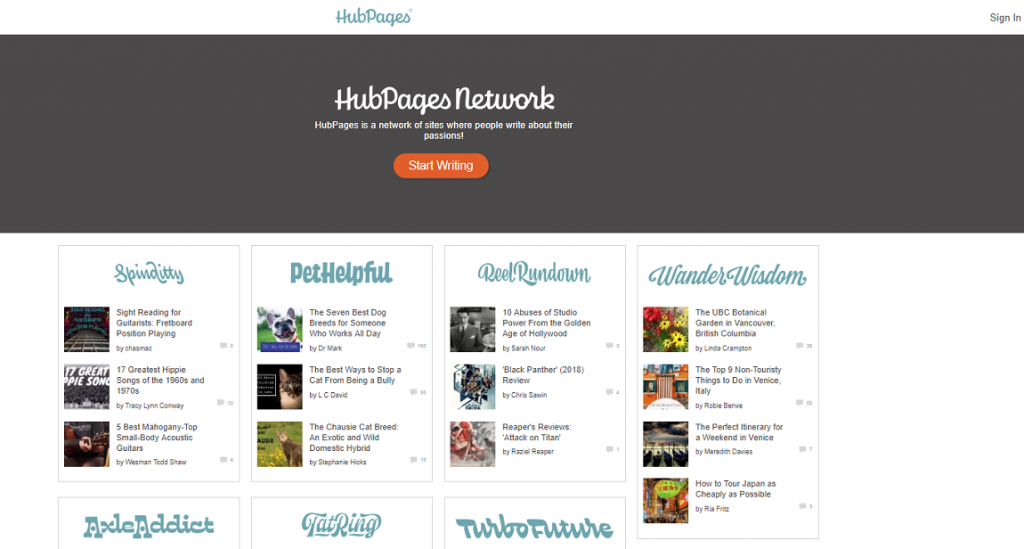This is a screenshot of the Hub Pages website. The top bar is white, with the Hub Pages logo slightly off-center towards the left. On the right edge of this bar is the "Sign In" option. Below the top bar, a semi-large gray rectangle features the Hub Pages network logo in semi-cursive writing. Underneath the logo, in a smaller, regular font, the text reads: "Hub Pages is a network of sites where people write about their passions." Further down, there is an orange oval-shaped button labeled "Start Writing" in white text.

The page is divided into various sections and categories, each outlined by thin gray lines. The first category on the left is "Spendiddy," which contains three groups. Adjacent to it is "Pet Helpful" with three links as well. Other categories listed on the page include "Real Rundown," "Wonder Wisdom," "Axle Addict," "Tat Ring," and "Turbo Future." These categories showcase different writings available on the Hub Pages network.